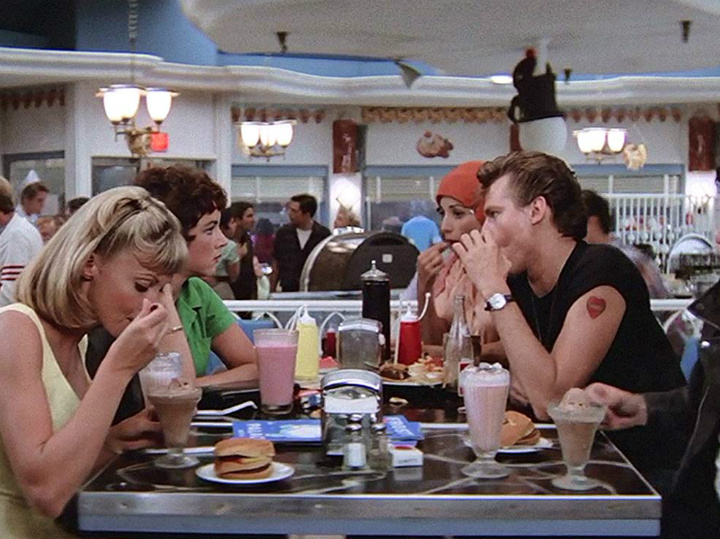This detailed still image is from the classic movie "Grease." It captures a lively 1950s diner scene featuring five main characters seated at a dining booth. At the forefront, Olivia Newton-John, who plays Sandy, is identifiable by her short blonde hair with bangs and a yellow shirt, savoring chocolate ice cream out of a glass. Adjacent to her is Rizzo, portrayed by a character with short black hair and wearing a green top, sipping a pink milkshake. Opposite them is a tough-looking guy with a heart tattoo, who may be Knicky, and further to the right is John Travolta as Danny, partially visible in a black leather jacket, also indulging in chocolate ice cream. Another female character in the background dons a red cap. The table is laden with milkshakes, burgers, and other diner fare, suggesting they are deep in conversation. The background brims with typical period details: a white wall, a jukebox, bustling servers in white hats, chandeliers, and windows on the back wall, all contributing to the retro ambiance of the iconic scene.